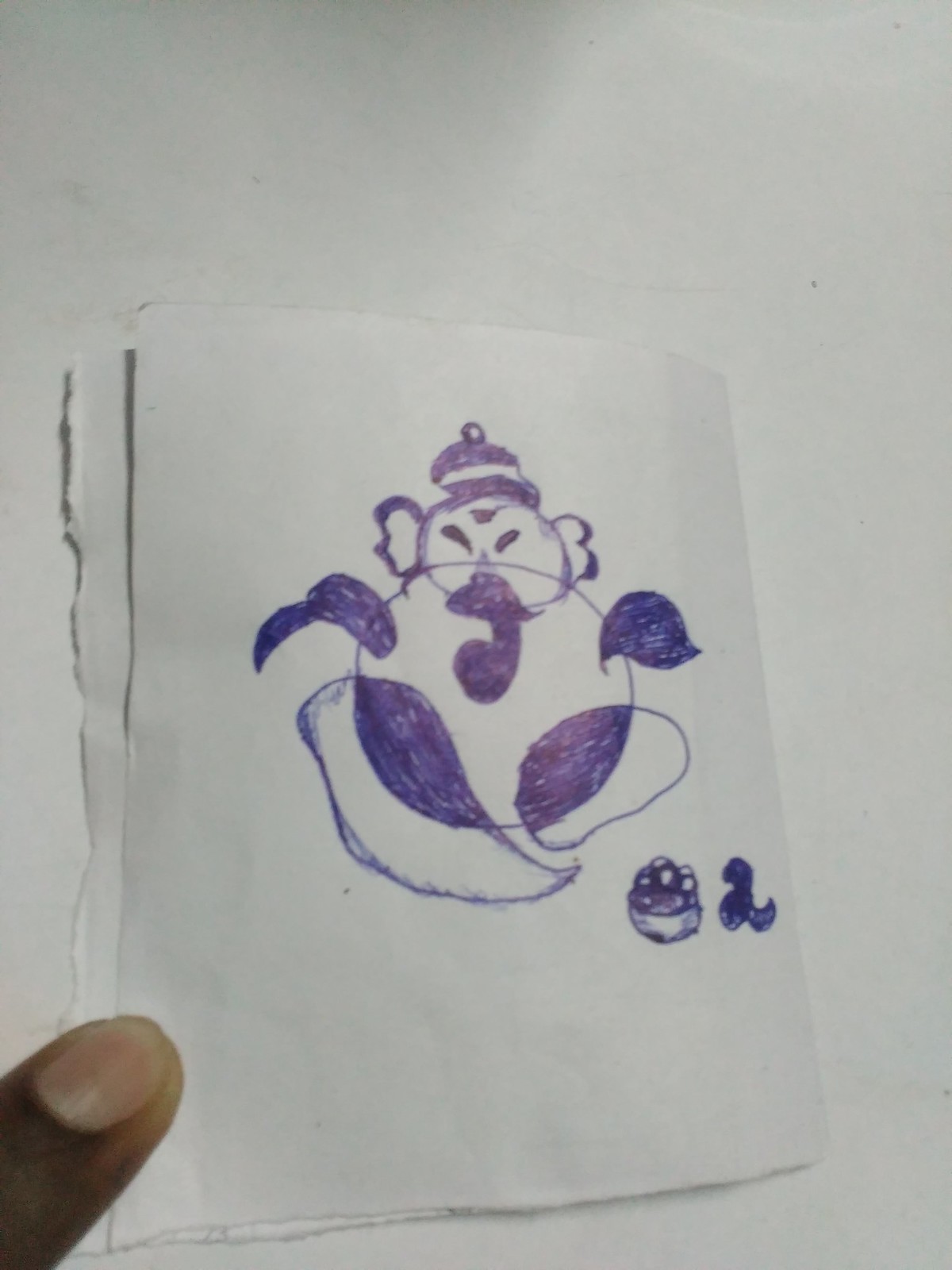This detailed photograph showcases a small piece of hand-drawn artwork on a folded piece of white paper. Rendered meticulously in blue pen ink, the illustration features a character reminiscent of a genie. The character is composed of a central circle representing the head, adorned with large ears and what appears to be a hat. From this head extends a set of swirly, arm-like shapes, and beneath them are folded, leg-like forms. The paper is gently held in the photograph by someone's fingertip, with their fingernail visible, resting against a smooth, white background. The composition captures the delicate and whimsical nature of the drawing, while the contrasting blue ink against the white paper creates a visually striking effect.